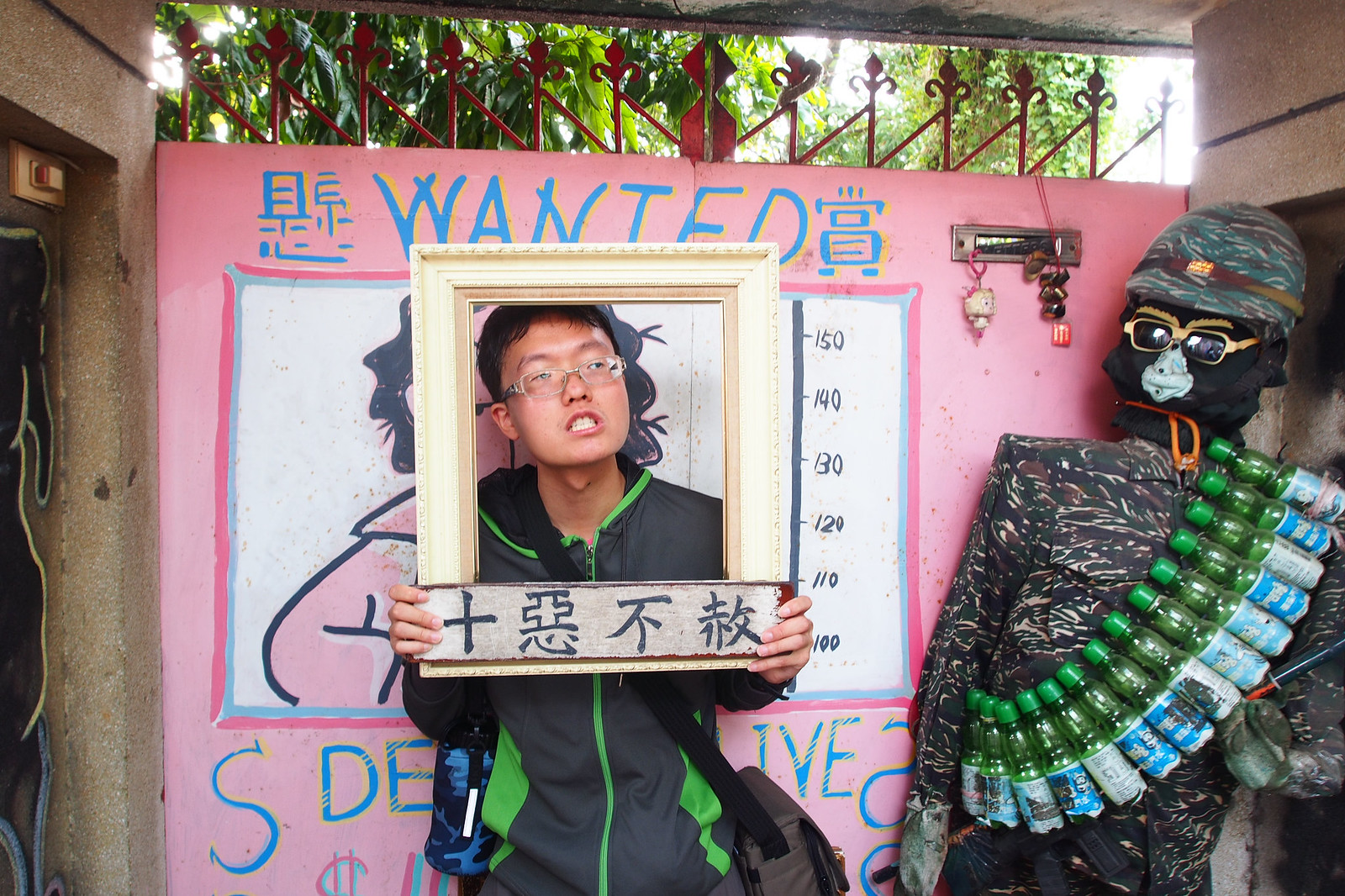The image captures an Asian man standing outdoors in China, likely in the middle of the day, holding a picture frame with Chinese lettering around his face. He is looking towards the camera, but not directly at it, and is grimacing. The man, wearing glasses and a dark jacket with green detailing, stands at the center of the image. He is in front of a wall with an English poster that reads, "WANTED: DEAD OR ALIVE," which partially covers a drawing of a person. To his right is a mannequin dressed in a military uniform, complete with a belt resembling an ammunition belt, which holds several liquid bottles on its chest. In the background, there is a gate and some vegetation, including trees, visible at the top of the image. The scene features various colors such as black, brown, green, pink, light blue, yellow, white, red, and maroon. The overall setting has the appearance of being within a photo booth setup.